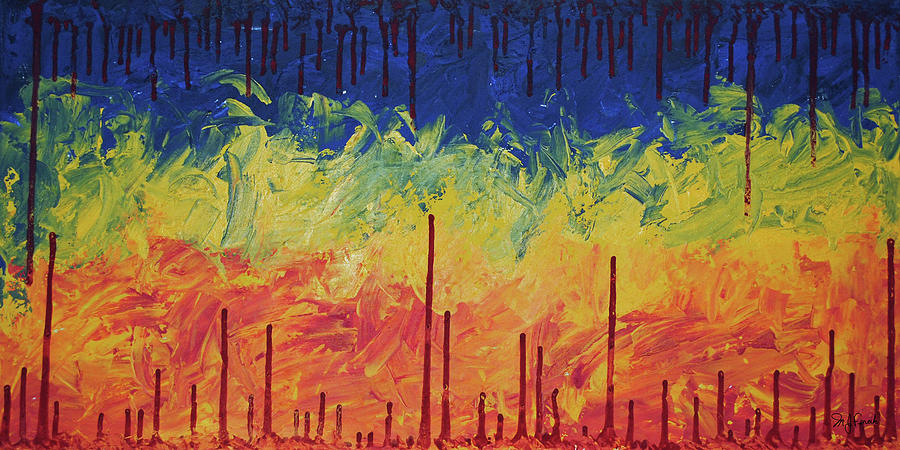This image depicts a wide, horizontal painting characterized by a striking use of color and abstract elements. At the very top, the painting features a dark blue background that fades into vibrant swirls of green and yellow in the middle. The transition between the colors is smooth, suggesting the artist may have used techniques like finger-painting or swirling with a brush. Towards the bottom, the painting shifts to vivid hues of red and orange. 

Prominent in the composition are the dark red paint drips that run from both the top and bottom towards the center, adding a chaotic and dynamic visual effect. These drips resemble tree trunks or streaks of paint that have been deliberately allowed to flow, hinting at a method where the painting was possibly turned upside-down during its creation. The overall effect might evoke the intense imagery of a forest fire, abstractly represented through the swirling colors and dripping lines. There are no discernible objects, people, or text within the painting, allowing the viewer to interpret its rich color palette and abstract form freely.